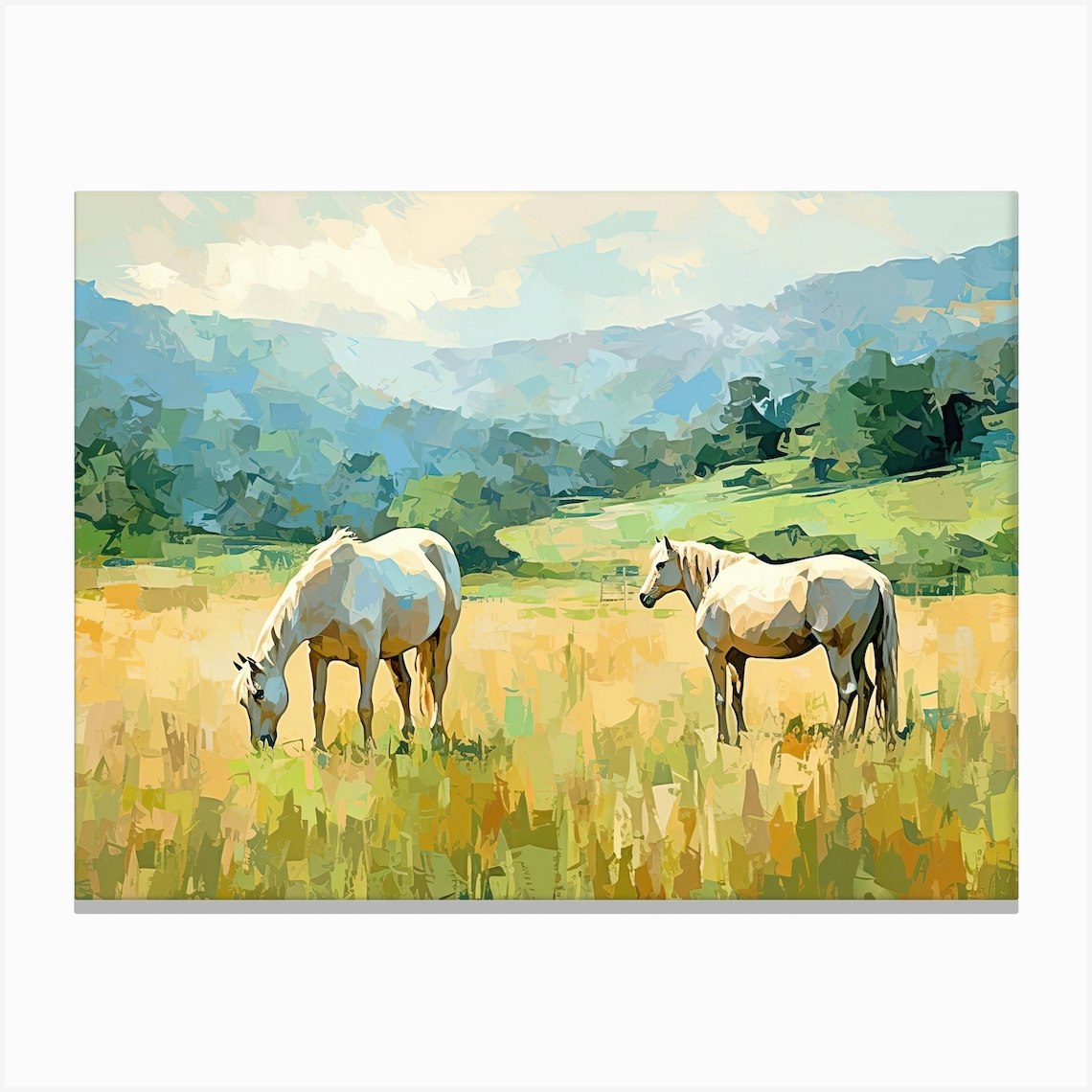A captivating, block-style painting illustrates a pair of wild, white horses in a mountainous pasture. The minimalist, unrefined brushstrokes convey a rustic charm, with one horse standing alert, gazing towards the distant mountains, while the other lowers its head to graze on the greenish-brown grass indicative of fall. The uneven, earthy tones of the mountain range in the background are punctuated with patches of white, hinting at snow-covered peaks. In the foreground, sprawling fields of grass transition from green to brown, dotted with large boulders, leading the viewer's eye to the rugged mountains beyond. The scene perfectly captures the untamed spirit of these majestic creatures in their natural, wild-west habitat.